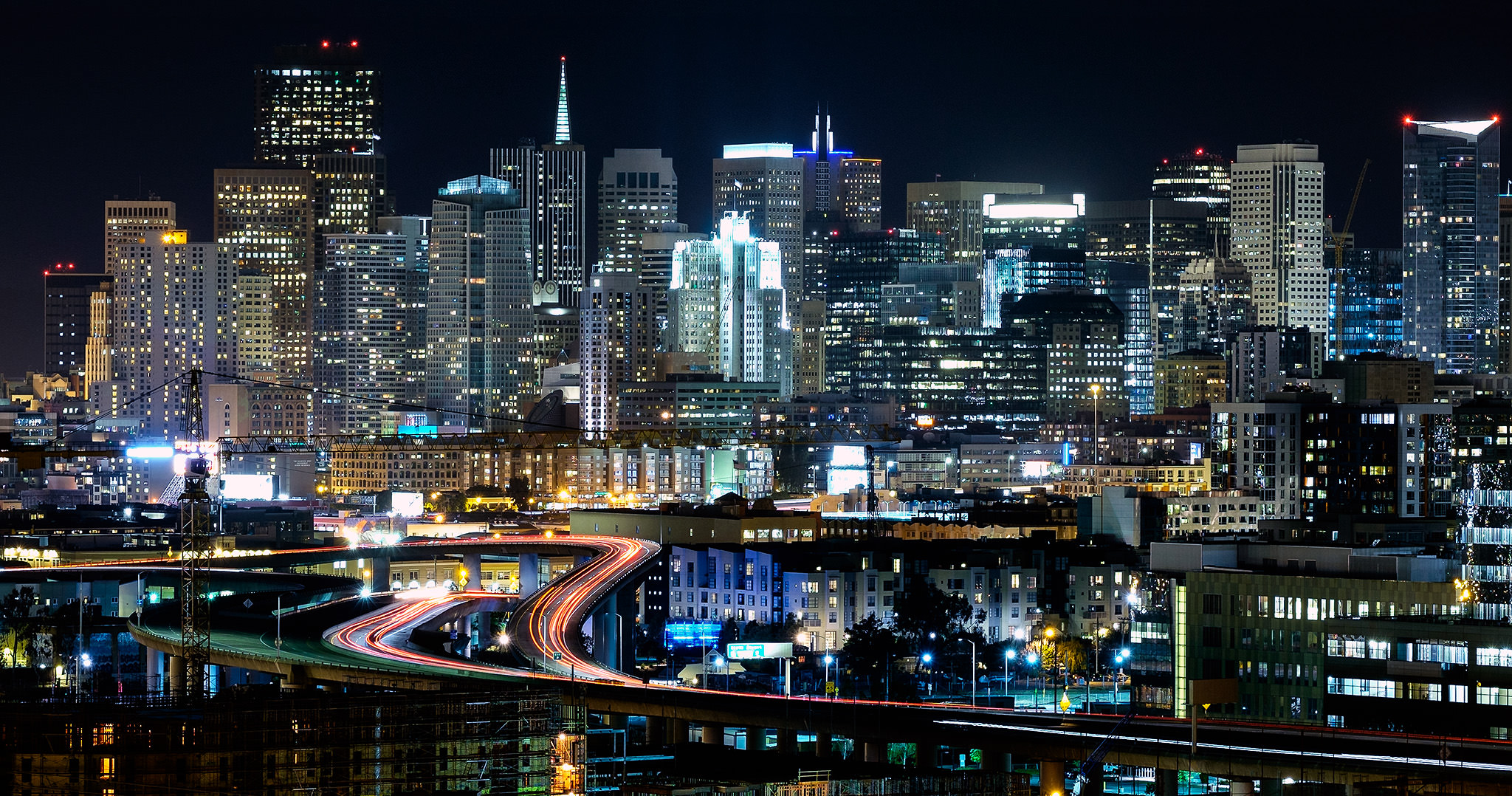The image captures a vibrant cityscape at night, showcasing a plethora of skyscrapers of varying heights stretching across the scene from left to right. The skyline is brilliantly lit with countless white, blue, and gray illuminated buildings, some adorned with red lights at their peaks. The entire scene is set against a backdrop of a solid black sky, devoid of stars or a visible moon.

In the foreground, a network of interweaving highways curves around, casting a reddish or rose-colored glow—likely from the headlights of moving cars—against the dark pavement. These highways appear to cross bridges and wind over a body of water at the bottom of the image. The water surface reflects the shimmering lights of the buildings and streets, creating a dynamic interplay of colors.

The bustling atmosphere is further emphasized by neon-like yellow and green lights seen on the roads, street signs, and the blurred streams of light from passing cars. In the distance, a train with visible green lights adds an extra layer of dynamism to the scene. The busy, cluttered nature of the city is palpable, making it feel alive and vibrant. Although the city is unidentified, its lively energy and the architectural diversity of its buildings—possibly including iconic structures like the Empire State Building—suggest a major metropolitan area, potentially even New York City.